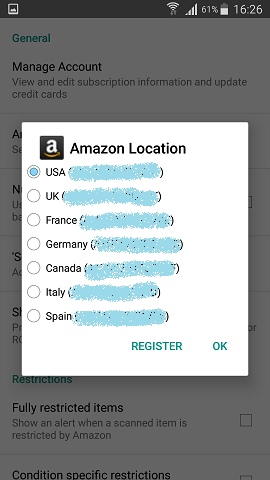This is a detailed screenshot of a smartphone taken at 4:26 PM, with the battery at 61%. The screen displays a section labeled "General," where options include "Manage Account," "View and Edit Subscription Information," and "Update Credit Cards." Overlaid on this section is a white box featuring the Amazon logo and labeled "Amazon Location." The box lists several countries—USA, UK, France, Germany, Canada, Italy, and Spain—with the USA being the only selected option. At the bottom right corner of the box, there are two buttons: one green button labeled "Register" and another labeled "Okay."